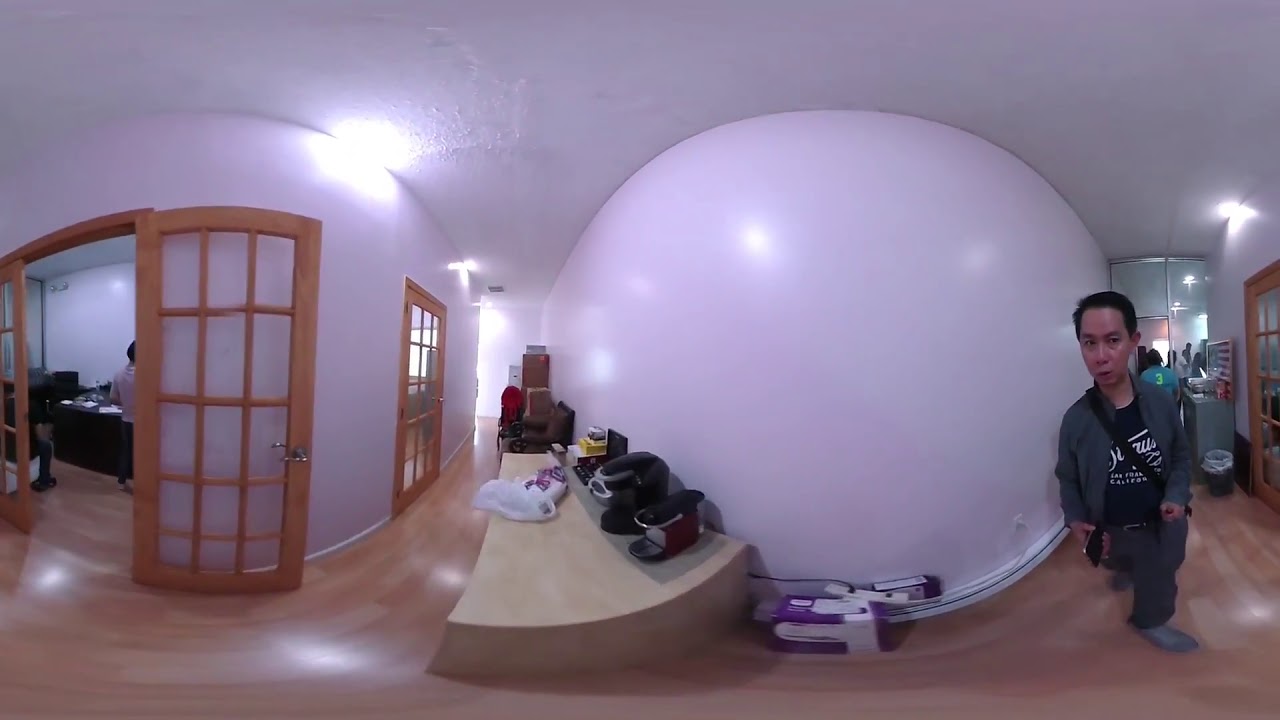This distorted image features a room where all the straight lines appear curved, giving objects a warped, circular appearance. On the right side stands a man of possibly Asian descent, facing the camera. He has short black hair and light brown skin. His eyes are open, and he wears a black t-shirt with white text, mostly obscured by a dark gray vest. A black crossbody bag is strapped across his chest, running down to his opposing hip. He also wears dark gray slacks and matching shoes. His hands just peek out from his jacket, and he holds a cell phone in his right hand.

Directly behind the man is a distorted, white, bubble-like shape created by the room’s warped lines. The floor, affected by the same distortion, is a polished, light brown wood. To the left, the wall, light purple in color, bulges outwards due to the special effects, giving it a ballooned look. The ceiling is covered in white stucco, with a bright light on the left side reflecting off it and part of the wall.

Beneath this light, on the far left are two wooden doors in a corner of the room. The leftmost door, characterized by several glass panels, is open, revealing a lit hallway. The other door closer to the center is closed. This corner, like other elements in the room, also appears to bulge outward due to the image’s distortion.

In the center of the image is a wooden platform holding a plastic white bag and some black and yellow items. Near the bottom center, there's a white, purple, and black box with a wire trailing around the distorted bubble shape towards the back. Over the man’s shoulder in the background, another person in a light blue shirt with a number three on the back is partially visible. The setting seems to be indoors, possibly during the day, giving an impression of an office setting.